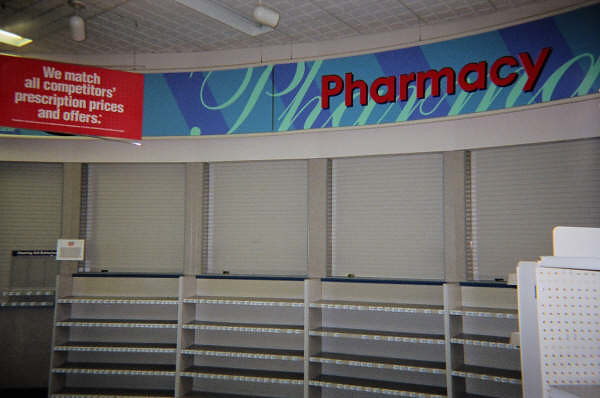The photograph depicts the front teller windows of a local pharmacy, which are currently closed. The windows are covered with shut metal bars painted white. At the top, there is a significant sign on a red background with bold white text, proclaiming, "We match all competitors' prescription prices and offers." To the right, a large banner displays the word "Pharmacy" in big red letters, with a larger cursive "Pharmacy" in white behind it. The background features a blue and dark blue striped pattern. Below these banners, there are barren shelves typically used to stock products; they are completely empty, devoid of items or price stickers. To the bottom right, an empty white pegboard stands uncluttered, with no products or labels. The walls of the pharmacy are a beige color, contributing to an older, somewhat dated design aesthetic. Security cameras are mounted to the ceiling, aimed in different directions, suggesting a focus on monitoring the area. The overall scene emphasizes the closed status of the pharmacy, with no activity or available merchandise visible.